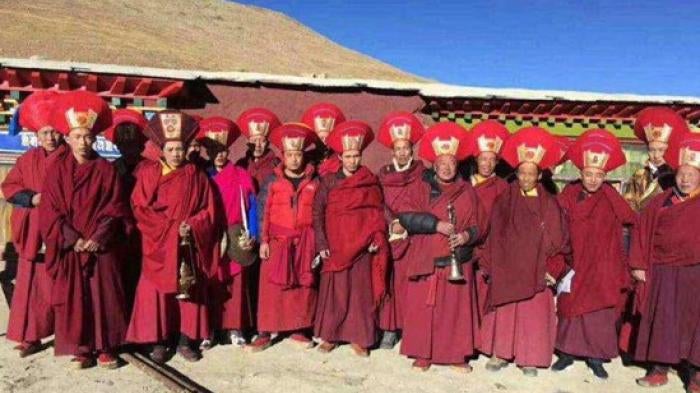In this aged and slightly blurry photograph, a group of around 20 men, most likely Chinese or Tibetan monks, are standing shoulder to shoulder, facing the camera on a sandy, earthy ground. They are dressed in ceremonial garb, each wearing a red robe that varies in shade from a lighter red to a richer burgundy. Their robes extend all the way down to their feet, complemented by matching red shoes. Each man is adorned with a distinctive, bright red hat that fans out widely on either side and rounds at the top, featuring a gold emblem or badge with a red mark centrally placed. A few men hold objects, including a lantern and a horn or trumpet. Behind them, a weathered building with a beige or light brown roof and hanging cloths with green, red, and black prints stands against a vibrant blue sky. The overall setting, with its earthy ground and contrasting backdrop, adds to the ceremonial and historical ambiance of the scene.